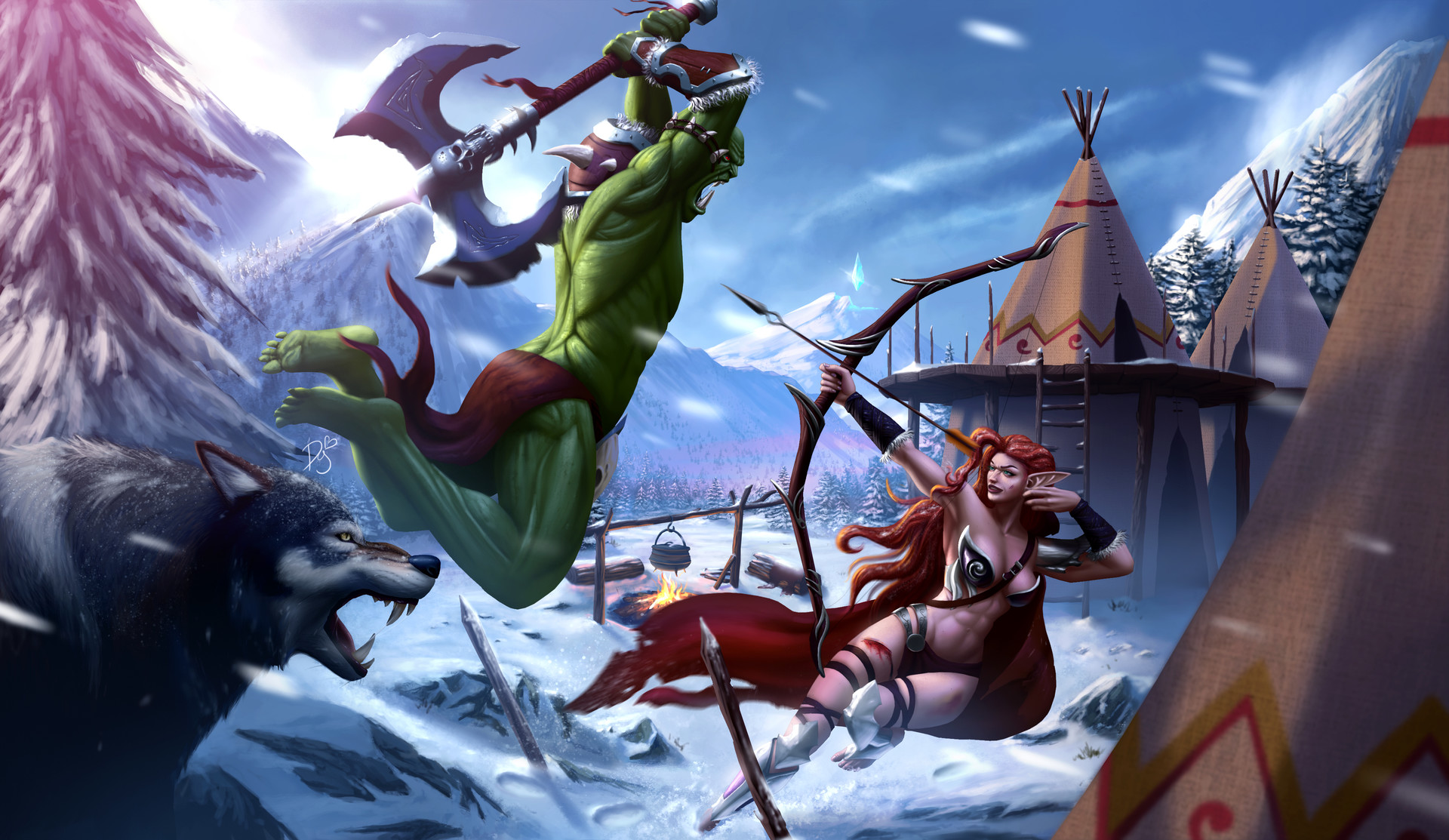In this detailed fantasy artwork, set against a snowy landscape, two fantastical characters are locked in an intense mid-air battle. Dominating the foreground is a hulking green orc-like creature, who wields a massive double-sided axe with a skull in its center. The orc, clad only in a red loincloth and some neck armor, has fierce long teeth visible and is poised to strike. Opposing him is a fiery-haired elven woman, who is scantily clad in black bikini armor adorned with leather straps and a flowing, tattered red cape. Her long, pointed ears and muscular figure are striking as she aims her bow and arrow directly at the orc. 

To the left of the battling figures, a snarling wolf with bared teeth is positioned before a snow-laden pine tree, adding to the tension of the scene. The background features a striking winter valley flanked by snow-capped mountains and dotted with pine trees. Centrally located in the image is a fire with a pot hanging over it, suggesting a recent camp. On the right side of the artwork, several large teepees, appearing to be two stories tall, stand tall on the snowy ground, further enriching the fantasy setting. The depiction is vividly detailed, creating a dynamic and immersive scene filled with action and intrigue.